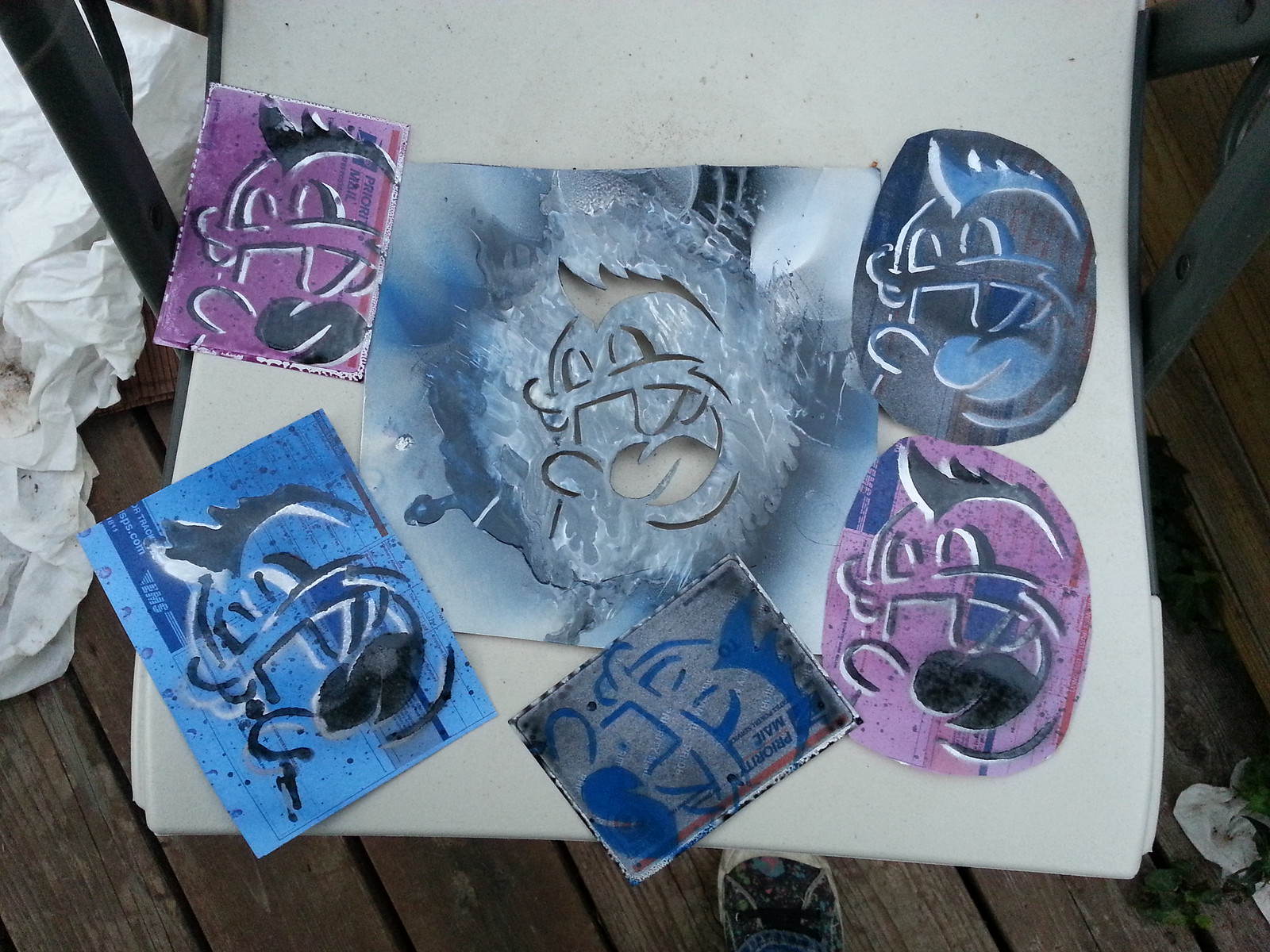The image showcases several airbrushed artworks on a piece of white cloth, which appears to be laid out on a wooden plank decking. The focal point is a cartoonish, animated character with fangs, a tongue sticking out, and a mohawk hairstyle. The character is spray-painted in various colors, including blue, light blue, dark blue, dark purple, and light purple. Surrounding the central incomplete stencil, which seems to serve as a template for further creations, are five completed pieces. These completed pieces have been cut into shapes like circles or squares. Notably, a few of these images are painted on what appear to be priority mail boxes or envelopes, with one having a blue background and black design, another with a gray background and blue design, and another with a black background and white design. Additional images feature a pink background. A sneaker, likely belonging to the person who took the photo, is visible at the bottom, and crumpled white paper lies to the left, adding to the artistic workspace atmosphere.